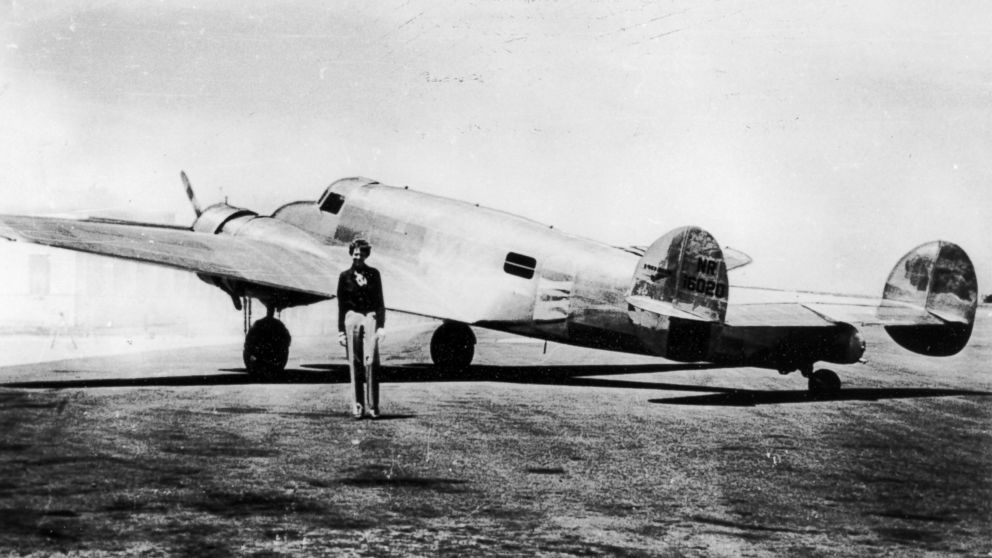This grainy vintage black and white photograph captures Amelia Earhart standing proudly in front of her all-metal airplane, model number NR16020, parked on a tarmac. Amelia, identifiable by her short hair and characteristic smile, is clad in a long black top and pants, presenting a stark contrast to the softer grayscale background. The imposing aircraft behind her boasts three visible wheels—two in the front, one in the back—along with its prominent wings and a single visible propeller. The image showcases one of the airplane’s cockpit windows near which Amelia is standing. The scene is backed by a sky that blends seamlessly into the grayscale tarmac, making the metallic sheen of the plane and the faint shadow it casts subtly stand out. Despite the graininess and age of the photo, the powerful presence of Earhart and her aircraft is unmistakable.